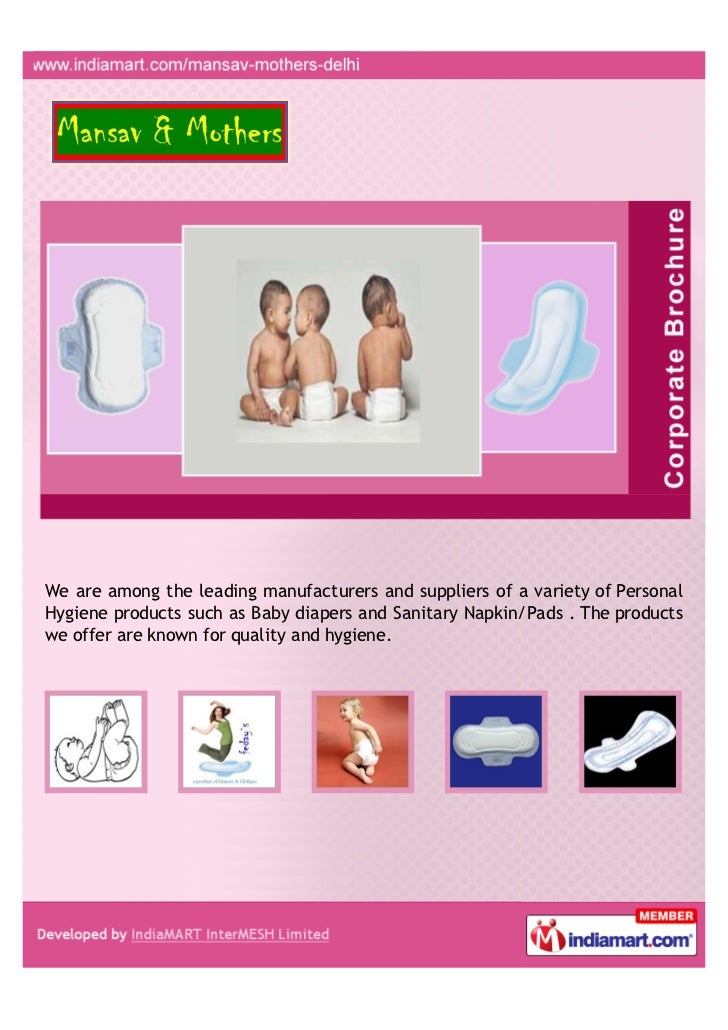This advertisement from IndiaMART.com, titled "Mansav and Mothers," features a corporate brochure for personal hygiene products set against a pink background with a subtle diamond design and darker pink stripes at the top and bottom. Prominently displayed in the center are three babies in white diapers; two of the babies are interacting with one another, their backs facing the camera, while a third baby sits forward, sucking his thumb and looking to the right. These babies are arranged in a row, flanked by two different-sized maxi pads on either side—one on the left and a larger one on the right, next to text reading "Corporate Brochure" in white.

Below the central image, there is textual content stating: "We are among the leading manufacturers and suppliers of a variety of personal hygiene products such as baby diapers and sanitary napkins/pads. The products we offer are known for quality in hygiene." Accompanying this message are additional images: a black and white clip art of a baby laying on its back, an animated image of a woman jumping to demonstrate the leak-proof quality of the maxi pads, another baby in a diaper, and two more maxi pads. The advertisement is part of IndiaMART.com, as noted in the lower right-hand corner. The color scheme used throughout is vivid and primarily consists of pink, red, white, and accents of green in the title box at the top, enhancing the overall visual appeal.